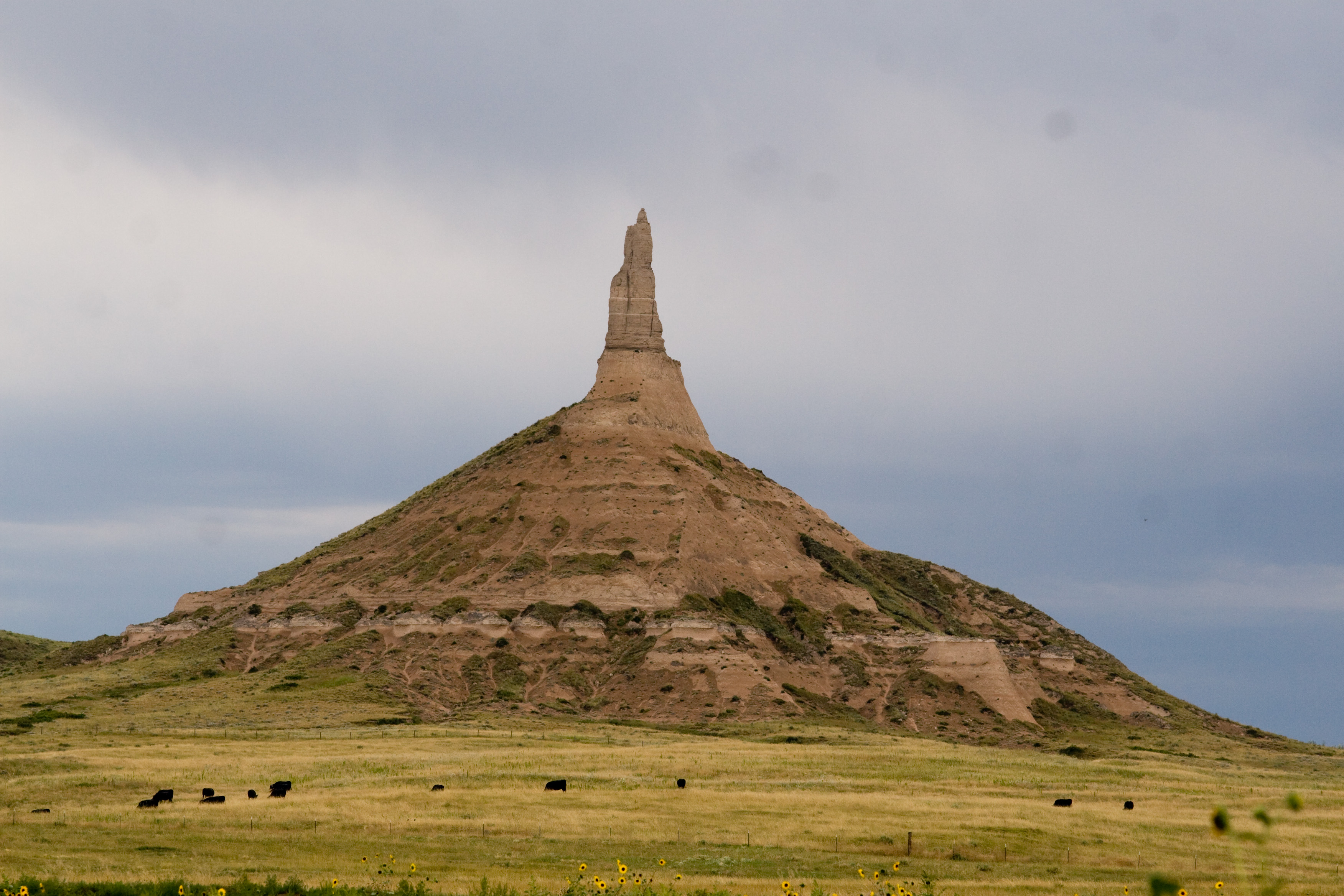The photograph captures an expansive green field scattered with dark brown and black cattle, concentrated mainly on the left side with a few stragglers in the center and right. This lively grassland, featuring shades of green and tan, stretches towards a grand hill in the distance. The hill is notable for its steep, rocky slopes comprising various shades of brown and sparse green vegetation. Rising sharply from the top of the hill is a distinct, cylindrical rock formation that resembles an old volcano with a pointed peak reaching into the overcast, bluish-gray sky, suggesting the possibility of rain. The scene is an intriguing blend of natural elements, showcasing the grazing cattle beneath the dramatic geological feature that stands as the focal point of the image.